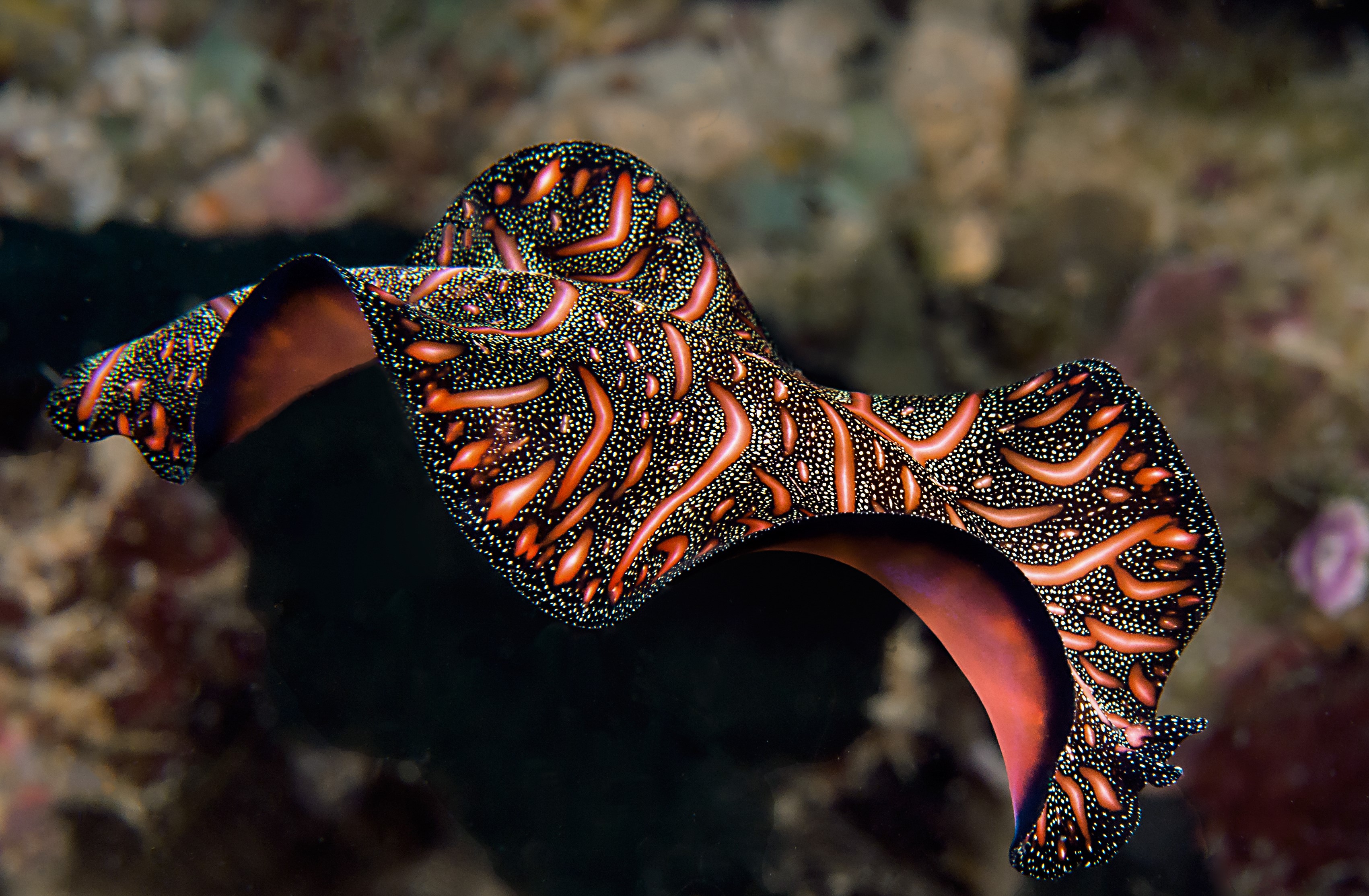This full-color photograph, primarily emphasizing an outdoor, underwater setting, captures an extraordinary and highly colorful marine creature swimming amidst an out-of-focus background of rocks and varied vegetation. The horizontally rectangular image showcases a unique, unidentified sea animal, characterized by its predominantly black body adorned with small white dots. Adding to its striking appearance are bright, tube-shaped patterns in shades of orange and white, interspersed across its form. These lines vary in length and thickness, enhancing the creature's almost ribbon-like, fluttering movement through the water. Underneath, where parts of its body flip upwards, the edges appear black, transitioning into a mottled orange and purple underside. Despite its worm-like and tent-like body structure, the creature's exact form remains ambiguous—evoking comparisons to a strange, beautiful flatworm or even an artistically rendered stingray, making it a mesmerizing subject in this vivid underwater scene.